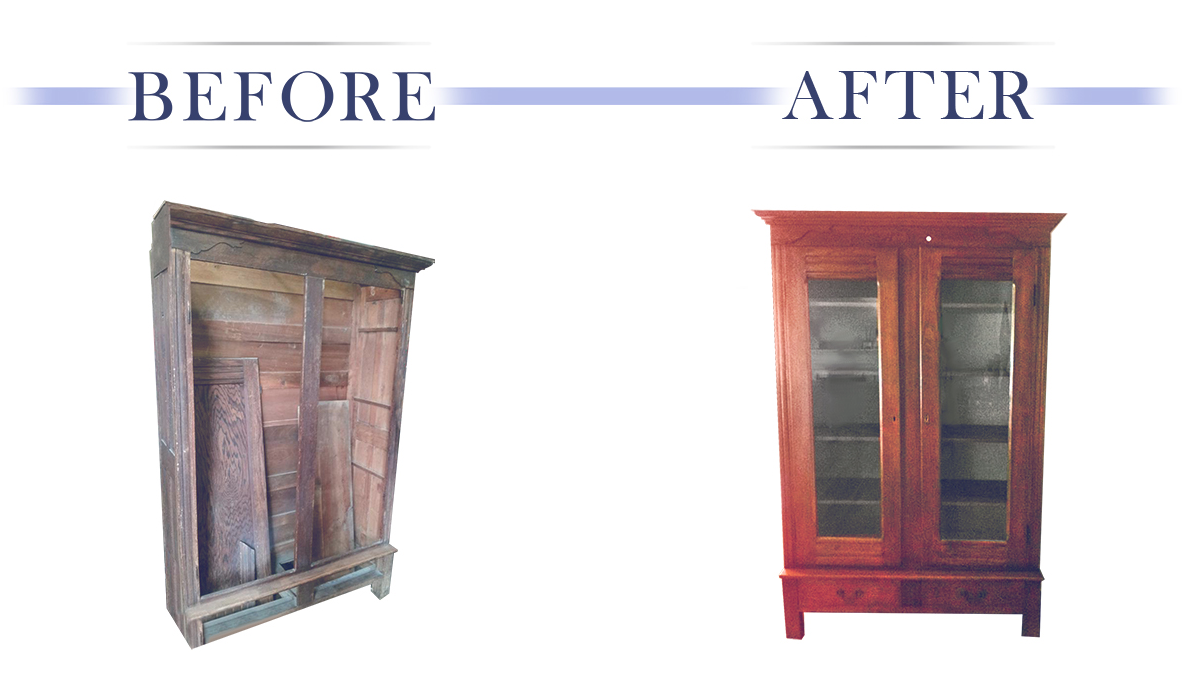The image shows before and after pictures of a restored upright display cabinet with glass doors, arranged vertically with the text "before" on the left and "after" on the right. The before picture reveals a weathered outer shell with fragments of doors and shelves inside, positioned against a white background. A faint violet line separates the images. The cabinet appears light wood and disassembled, presenting a faded, rickety appearance. In contrast, the after picture showcases a meticulously restored cabinet, finished in a beautiful mahogany or amber wood stain with locking glass doors, two drawers underneath, and five sets of shelves. The interior of the cabinet, now complete with a decorative greenish-gray background, exhibits an elegant and polished look. The transformation highlights the craftsmanship and care taken to revitalize the cabinet, turning it into a stunning and functional display piece.